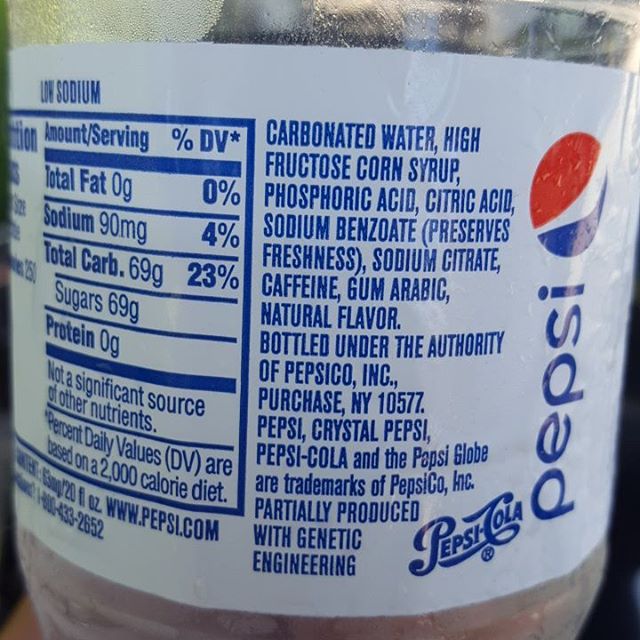This image captures the back of a clear plastic Pepsi bottle. Dominating the right side of the bottle is the iconic Pepsi label, featuring the word "Pepsi" in bold, blue text. Below this, the classic Pepsi-Cola logo is showcased in an elegant, curly script. The label is predominantly white with blue text, giving it a crisp and clean appearance. The circular Pepsi logo, recognizable by its blue, white, and red colors, is also prominently displayed, complete with its signature wave design.

Though the Nutrition Facts panel is partially visible, only the right column can be seen, rendering some information cut off. The focus of the image is on the ingredients list, beginning with carbonated water and high fructose corn syrup, and continuing with other components typical of a soft drink. The bottle appears to be photographed in an indoor setting, possibly under artificial lighting during the daytime, but the background is indistinct and does not offer any particular details.